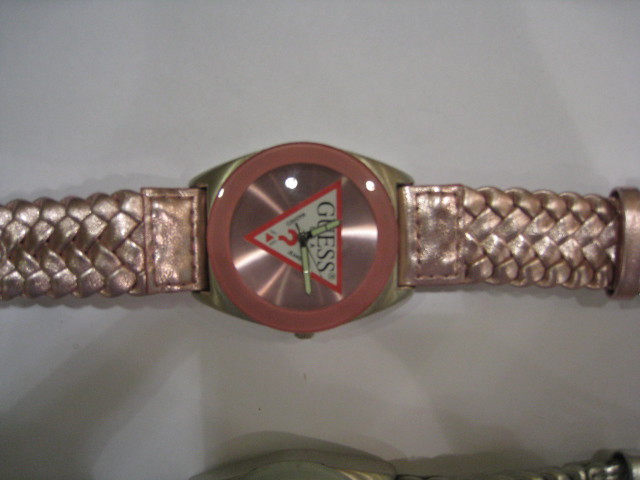In this image, we observe a photograph being taken of a watch positioned on a table. The shadows cast reveal the presence of hands and a head, likely belonging to the photographer. Central to the image is a prominently displayed watch, which is evidently the primary subject of the photograph. However, tucked at the very bottom of the frame, another watch makes a subtle appearance, laying flat on its side.

The focal watch features distinctive design elements—a striking upside-down triangle with a point directed downward, showcasing the word "GUESS" at the top of the triangle and a red question mark below. The watch face eschews traditional numerical markers or lines, emphasizing its minimalist design, which aligns with the playful "GUESS" branding. The hands of the watch are centrally placed within the triangle, further contributing to the enigmatic theme suggested by the absence of markers.

The face of the watch boasts a refined rose gold hue, encased in a complementary gold-colored bezel. This elegant timepiece is paired with rose gold leather straps, creating a cohesive and stylish appearance. The overall composition of the photo, coupled with the intricate details of the watch, highlights its sophisticated yet intriguing aesthetic.